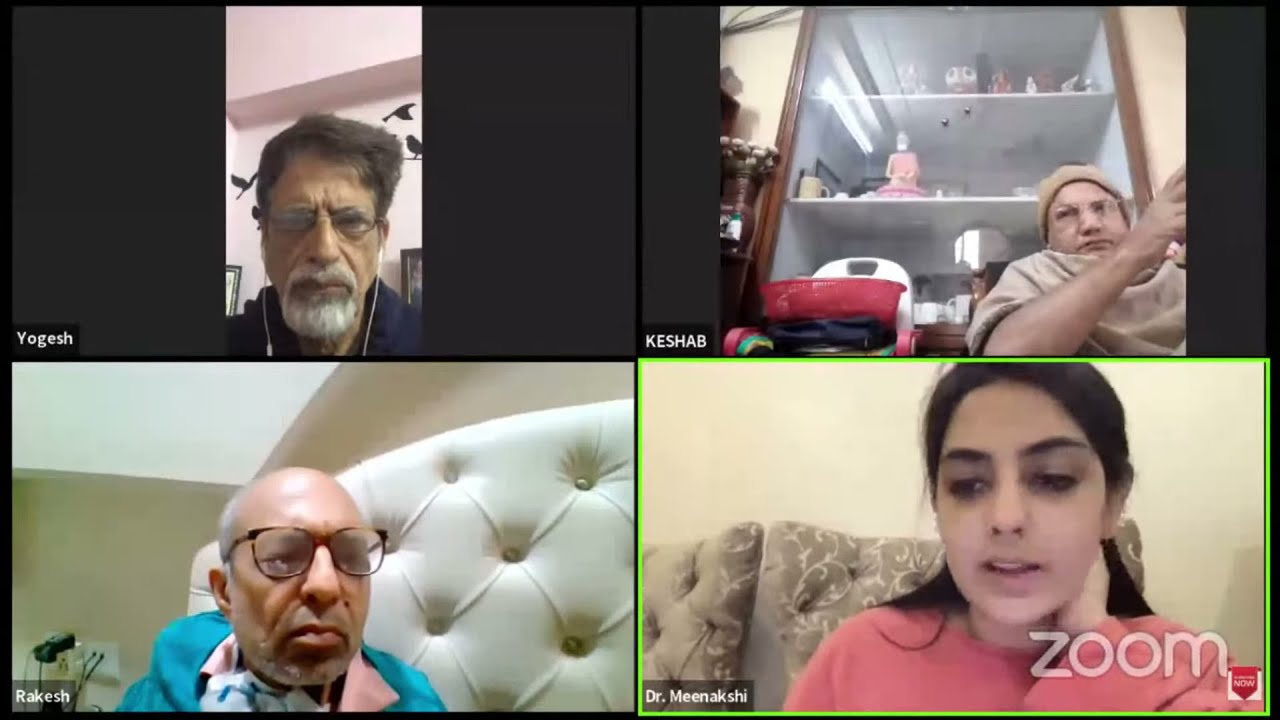This image is a detailed screenshot from a Zoom call featuring four participants. Positioned in the upper left quadrant is Yogesh, an older man with dark hair, wearing glasses and sporting a white goatee. In the upper right, we have Keshav, seated in front of a bookshelf or curio cabinet, dressed in a beige shirt and a beige hat, also wearing glasses. The lower left shows Rakesh, comfortably seated in a large padded white leather chair within a beige room; he is an older, bald man wearing glasses. Finally, in the lower right corner is Dr. Meenakshi, a woman with dark, pulled-back hair, wearing a pink shirt, seated on a beige chair with a white floral pattern against an off-white wall. In this moment, she appears to be speaking while the other participants listen attentively. The Zoom logo is visible in the lower right corner of the image, and there are no other interface elements or text present.